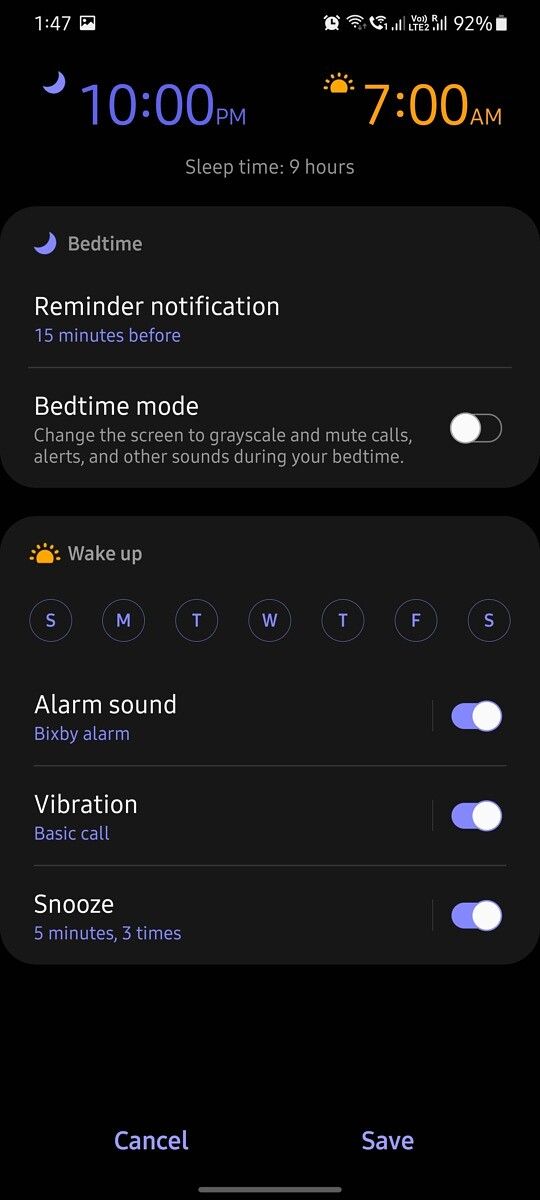The image is a detailed screenshot of a smartphone's alarm and bedtime settings interface. The time displayed on the phone is 1:47 PM, with the Wi-Fi signal and carrier signal showing three bars and a battery life of 92%. An alarm is set for 10:00 PM, indicated in a blue font alongside a moon graphic, designating bedtime. 

On the right side of the screen, a label shows "Wake Up" next to a sun graphic set for 7:00 AM, suggesting a sleep duration of nine hours. The moon icon repeats where it mentions "Bedtime," also highlighted in blue. A reminder notification appears in white, set to notify the user 15 minutes before bedtime. 

There is a toggle for "Bedtime Mode" that will change the screen to grayscale and mute calls, alerts, and other sounds during sleep hours. The "Wake Up" label reappears with a sun graphic. 

A calendar shows the days of the week abbreviated in circles with blue text, listing Sunday through Saturday. The alarm sound is set to "Bixby Alarm" and the vibration for basic calls is enabled, both marked in blue.